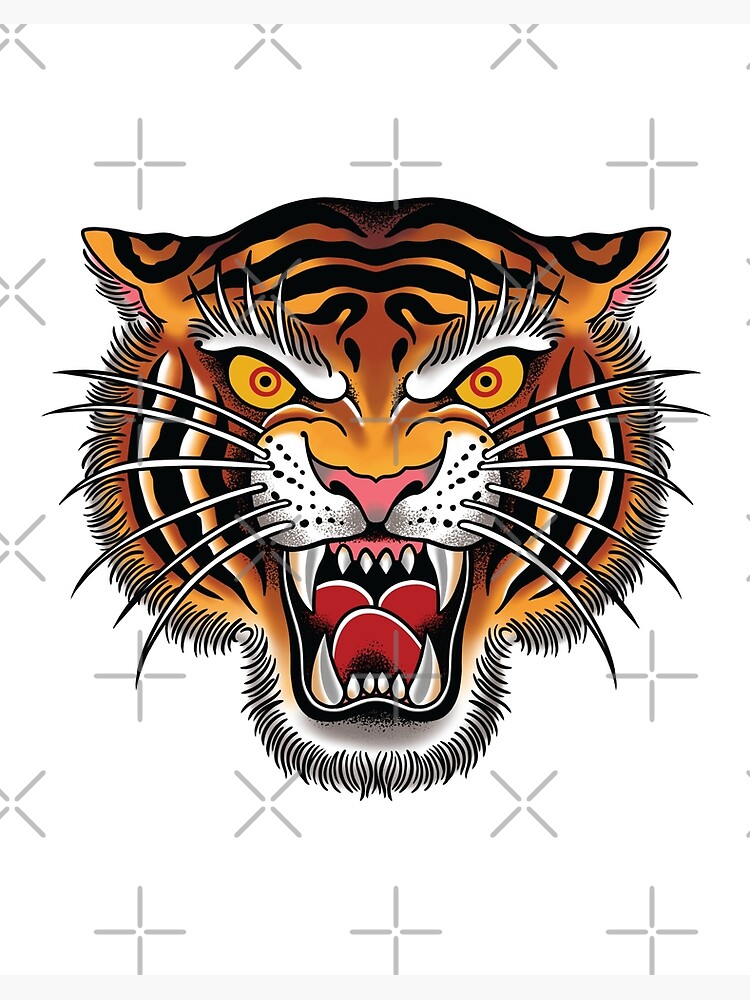This detailed digital artwork features an imposing Bengal tiger head, stylized with a blend of American traditional and tattoo designs. The tiger, predominantly orange with black stripes, is rendered in a meticulous drawing style, showcasing individual hairs, particularly white ones around the edges. Its face is ferocious, with a wide-open mouth revealing huge fangs and a prominent red tongue. The tiger's intense yellow eyes with red irises and black pupils glare menacingly, framed by big bushy white eyebrows. Notably, the tiger has six long white whiskers on each side of its pronounced nose. The white background is accentuated with light gray X's and crosses, resembling registration marks, which enhances the focus on the striking tiger face. The overall appearance of the logo conveys both a fierce and captivating expression, reminiscent of a traditional mascot yet bearing an almost dragon-like ferocity.